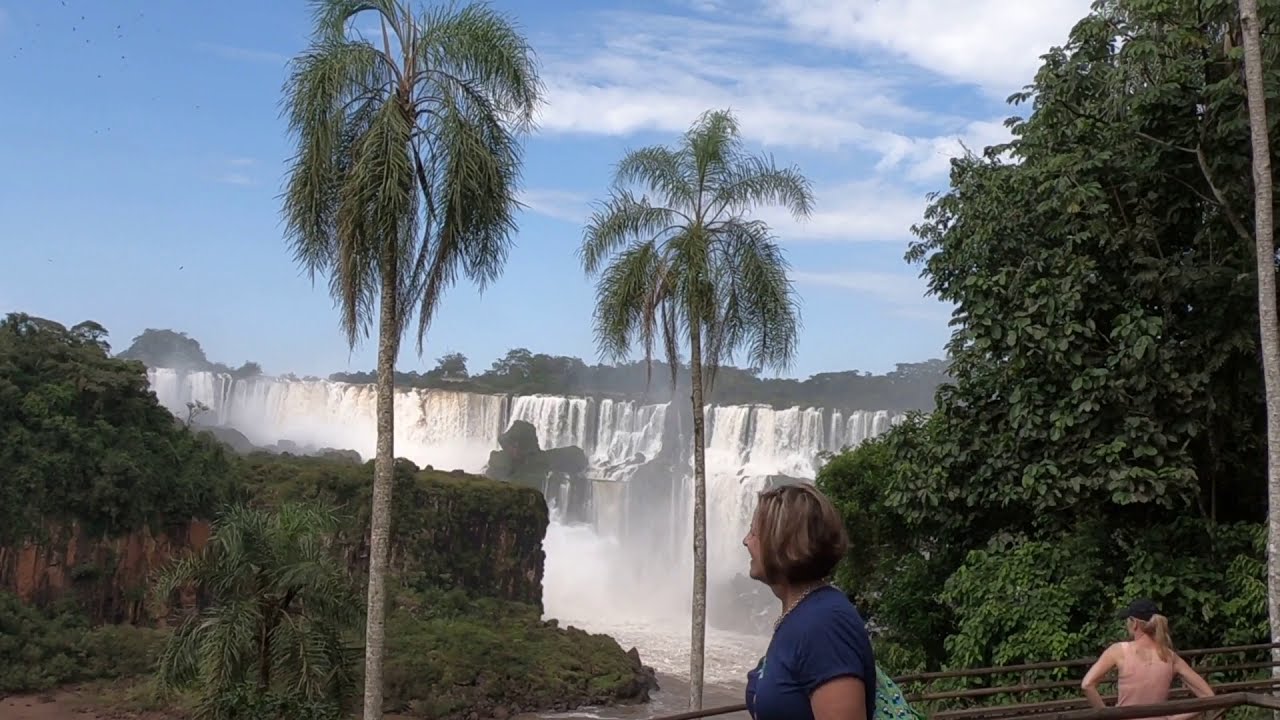The photograph captures a stunning landscape dominated by a large, majestic waterfall at the center and extending to the left and center-right of the image. White water cascades dramatically down, creating a misty backdrop that envelops the scene. In the foreground, two Caucasian women draw attention. On the right side is a woman with short, dirty blonde hair wearing a dark navy blue t-shirt, looking towards the center of the image. Beside her, with her back turned to the camera, stands another woman in a peach-colored tank top, black baseball cap, and blonde ponytail, her hands on her hips as she gazes at the waterfall.

Flanking the waterfall are two prominent palm trees, one situated about a third from the left and another near the center, both stretching upward with their leaves framing the upper part of the image. The left side also reveals a lush hillside adorned with green bushes and extending down to the bottom left corner. On the right, a bushy tree with abundant green leaves can be seen, contributing to the verdant scenery. Above, a partly cloudy sky transitions from clear blue on the left to clouds forming towards the top center, adding depth to the serene yet dynamic landscape.